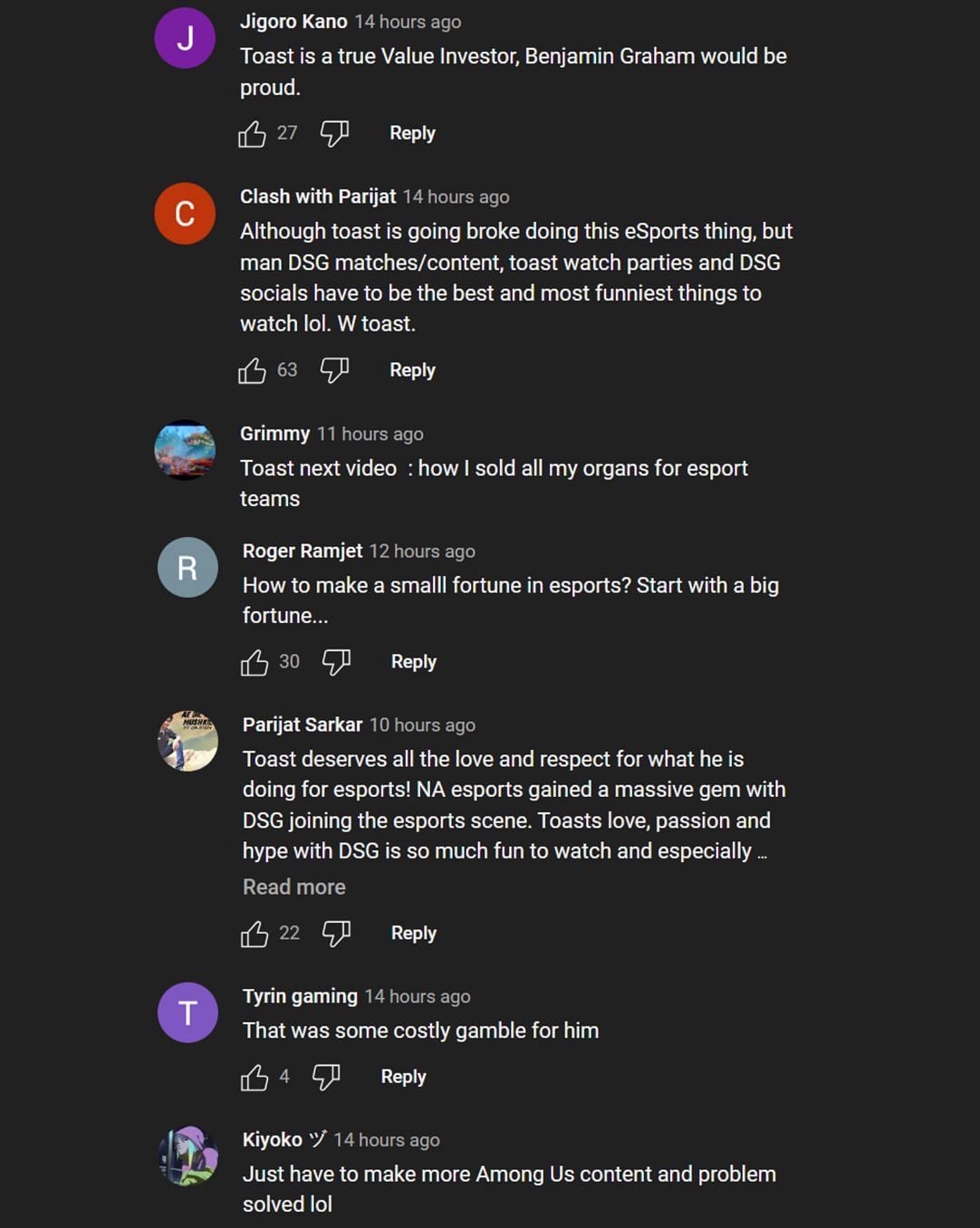### Descriptive Caption

The image features a stark black background with overlaid text depicting user comments and opinions about Toast's recent endeavors in eSports. At the top, prominently displayed are the letters "GIG over R" and below that, "KAAO," which may be acronyms or placeholders.

**Highlighted Comments:**
1. **Parajit (14 hours ago):** Toast, acknowledged as a true value investor, might have made Benjamin Graham proud, garnering six likes. Despite financial struggles in the eSports venture, the content from DSG matches, watch parties, and socials has been incredibly entertaining.
   
2. **Jimmy (11 hours ago):** With 63 likes, Jimmy humorously suggests the title for Toast's next video: "How I Sold All My Organs for eSports Teams."

3. **Roger Ramjet (12 hours ago):** Roger sarcastically comments on the financial risks of eSports, stating, "How to make a fortune in eSports: Start with a big fortune," receiving 30 likes.

4. **Panjit Setcar (11 hours ago):** Expressing admiration, Panjit notes that Toast has brought unparalleled love and respect to eSports. DSG joining the scene has been a major boost, making the content enjoyable to watch and read, with 22 likes.

5. **Tryin Gaming (14 hours ago):** Acknowledges the high risks involved in Toast's eSports investments.

6. **Kojo (14 hours ago):** Advises Toast to create more "Among Us" content as a solution to financial difficulties.

In summary, the comments reflect a mix of admiration, humor, and concern for Toast's bold venture into the eSports industry, highlighting its entertaining content and the community's supportive yet realistic outlook.